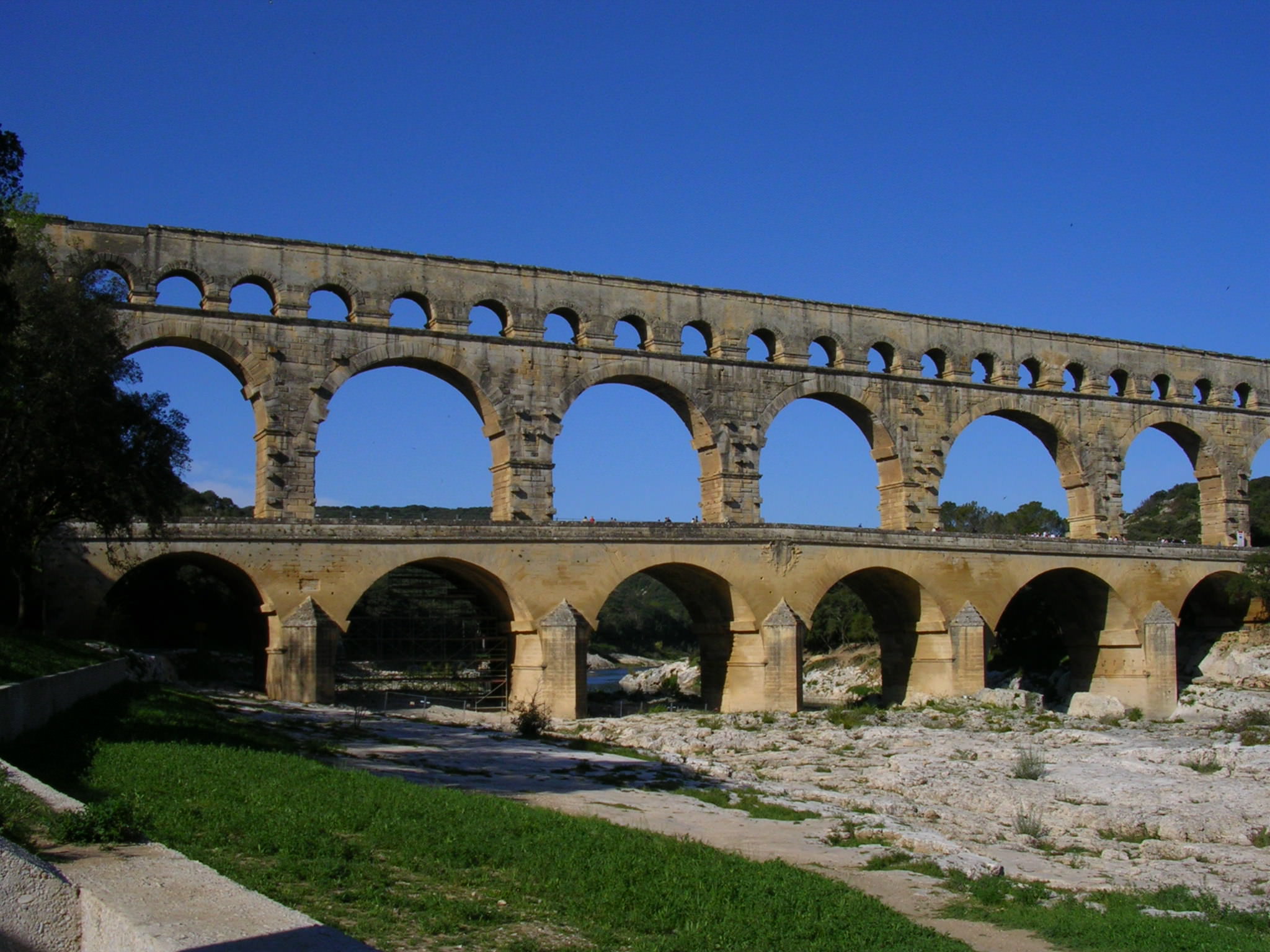The image captures a distant view of an ancient Roman aqueduct, exhibiting a multi-tiered series of archways. The structure features six large foundational arches at the bottom, supporting an additional set of six smaller arches above, and a final tier of even smaller decorative arches on top. Small figures can be seen walking, indicating the photo is taken from a considerable distance. The setting is on a bright, sunny day, with a clear, cloudless blue sky. The aqueduct, rendered in a faded tan due to centuries of wear and tear, stretches across a background of green trees and hills to the right. The left side of the image shows a tree and a dirt path, and in front of the structure, a mix of dirt and gravel can be seen, along with bits of green grass. There is an ongoing construction inside one of the lower arches, suggesting repair work on potential damage. The aqueduct's design, with its layered arches, not only exemplifies Roman engineering but also served historically significant functions, including the control of water flow and transportation.